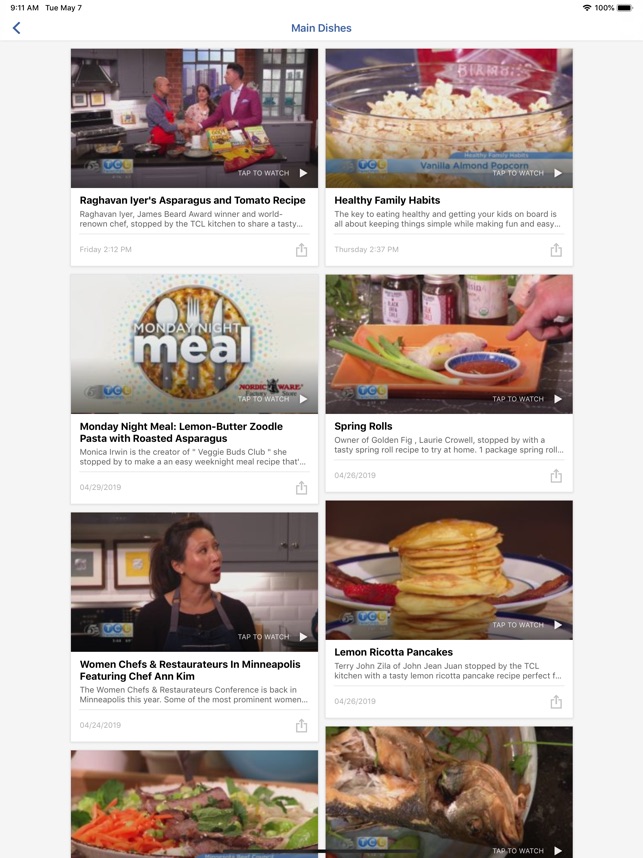Screenshot of a phone screen displaying a website focused on culinary content. The timestamp at the top reads 9:51 AM, Tuesday, May 7th, with a fully charged battery indicator at 100%. The main section of the screen is categorized under "Main Dishes," listing eight video thumbnails, each representing a different recipe.

Starting from the top left and moving clockwise:

1. An asparagus and tomato recipe, shown with a video thumbnail featuring a kitchen setting with a chef, potentially two hosts, and some cookbooks, indicating the chef may be promoting his cookbooks.
2. "Healthy Family Habits," displaying a bowl of vanilla almond popcorn.
3. A spring rolls recipe, illustrated by a spring roll with dipping sauce.
4. Lemon ricotta pancakes, depicted with a close-up image.
5. An unidentified chicken dish, without visible text.
6. A stir fry that appears to include pork, carrots, and assorted greens, shown without accompanying text.
7. "Women Chefs and Restauranteurs in Minneapolis," featuring an image of Chef Ann Kim.
8. "Monday Night Meal," with a video for lemon butter zoodle pasta with roasted asparagus.

Each thumbnail is designed to be clickable, leading to detailed video recipes for viewers to explore and enjoy.